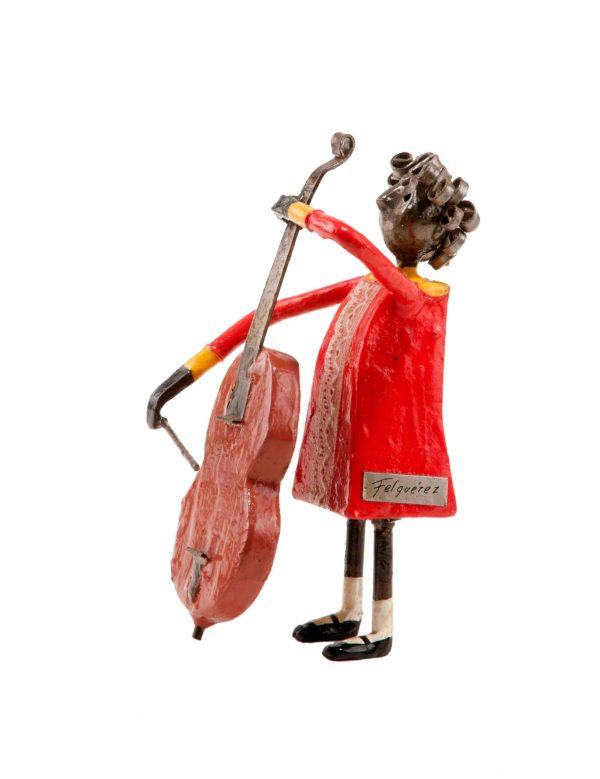The image depicts a detailed sculpture of a young girl playing the cello, seemingly carved from metal due to the dark, metallic sheen of her head and curly hair. She is dressed in a vibrant orange dress with yellow accents at the cuffs, and a full lace panel running from the neck to the hem. The figure stands erect, wearing white socks and black Mary Jane shoes. Holding the top of the cello with her left hand and a bow in her right, she appears poised to play. At the bottom left side of her dress, there is a gray rectangle with the inscription "Felgereth."